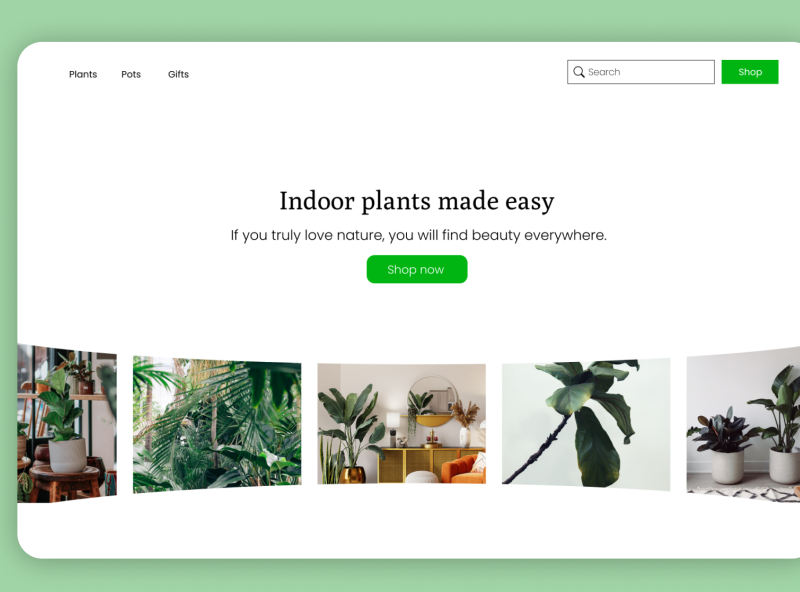This is a screenshot of a website showcasing indoor plants. The image appears to be of low resolution and is partially cut off on the right side. The screenshot is framed with green bars and has a white square in the upper left corner. Black text in the white square reads "plants, pots, gifs." At the upper right corner, there is a search field that features a black magnifying glass icon, and next to it, an orange rectangle with white text that says "Shop."

Centrally positioned, the bold black font headline reads "Indoor Plants Made Easy." Below this headline, in smaller black text, is the quote, "If you truly love nature, you will find beauty everywhere." Directly below the quote is another orange rectangle with white text that says "Shop Now."

Further down, there is a horizontal row of images depicting various potted plants. From left to right, the first image shows a white pot with a green plant. The next image is a closer view of a palm tree's top. Following that, there is a potted palm in a brass pot placed next to a stand with a mirror. The next image is a close-up of a branch with leaves. The final image shows two white potted plants placed on the ground.